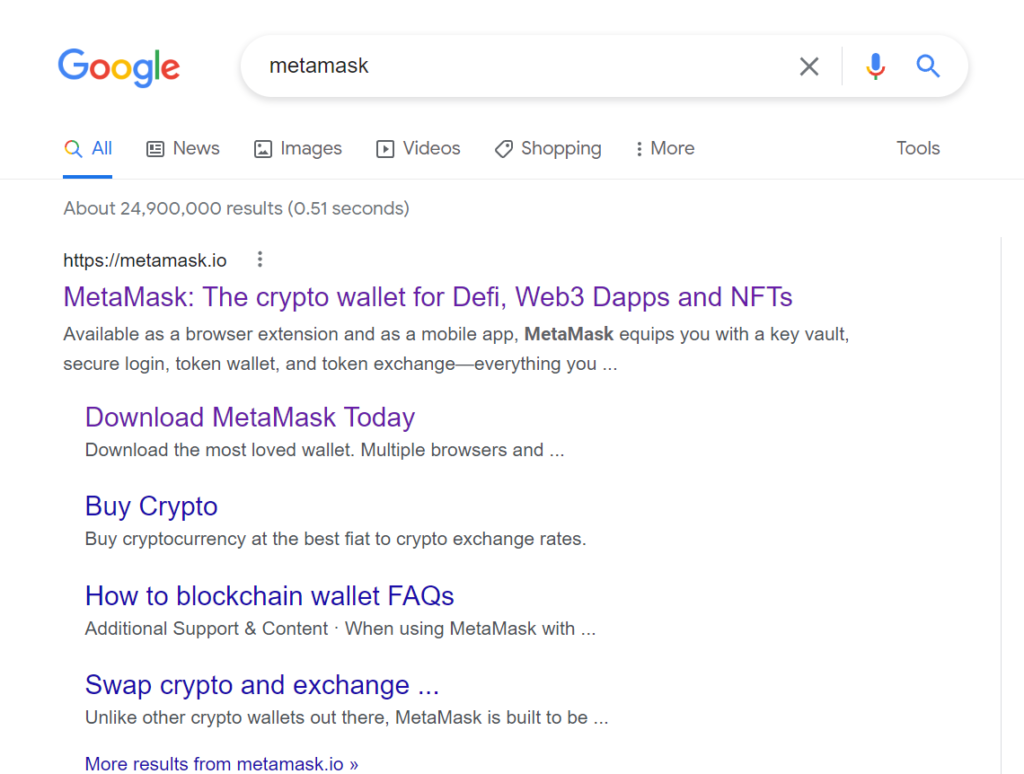The image on the homepage showcases a Google search results page for "MetaMask," highlighted at the top of the screen. The search term is clearly displayed, with "MetaMask" spelled out as M-E-T-A-M-A-S-K. The user is currently viewing the "All" section of the search results, with additional tabs for News, Images, Video, Shopping, and More. In small text beneath the search bar, it indicates there are approximately 25 million results.

The first search result shown is for MetaMask, titled "MetaMask – the crypto wallet for DeFi, Web3 dApps, and NFTs." This title appears in purple, suggesting the user has visited this link previously. The description underneath reads: "Available as a browser extension and as a mobile app. MetaMask equips you with key vaults, secure login, token wallet, and token exchange," with the words "MetaMask" and "equips you with" bolded for emphasis. The description also includes a prompt to "Download MetaMask today."

Additional hyperlinks are displayed below this description, including "Buy Crypto," "How to Blockchain Wallet FAQs," and "Swap Crypto," offering more specific guidance for users. The results are clearly marked as more from MetaMask in smaller text.

The search page features a white background with the colorful Google logo at the top left, adjacent to icons for voice search and a magnifying glass, all rendered in blue.